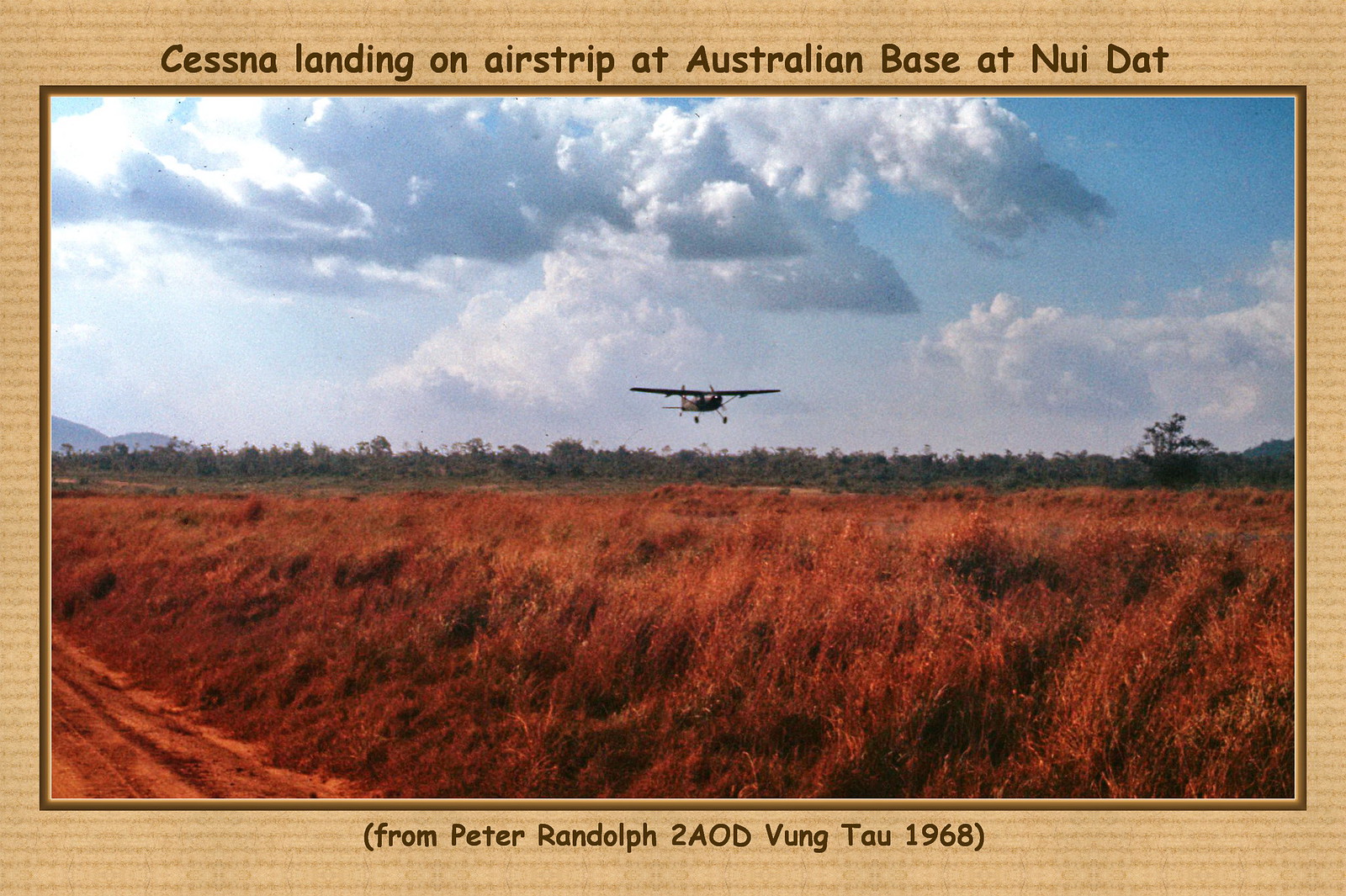This photograph, evocative of a vintage postcard from the Vietnam War era, captures a poignant moment at an Australian base at Nui Dat in 1968. It's a wide shot, beautifully split between a vast blue sky adorned with fluffy white clouds on the top half, and a reddish-orange field on the bottom half. The field, possibly covered with dead grass or wheat, extends towards a row of distant trees, adding depth to the landscape. In the lower left-hand corner, a portion of a muddy, orangey-brown dirt road is visible, suggesting minimal use. Dominating the center of the image is a twin-engine Cessna airplane, its wheels down, seemingly in the final moments before landing. This small aircraft, reminiscent of crop dusters, elegantly bridges the expansive sky and the earthy field below. The image is captioned at the top: "Cessna landing on airstrip at Australian base at Nui Dat," and below it, inscribed in brackets: "From Peter Randolph to AOD Vung Tau 1968," marking it as a historic relic from a bygone era.